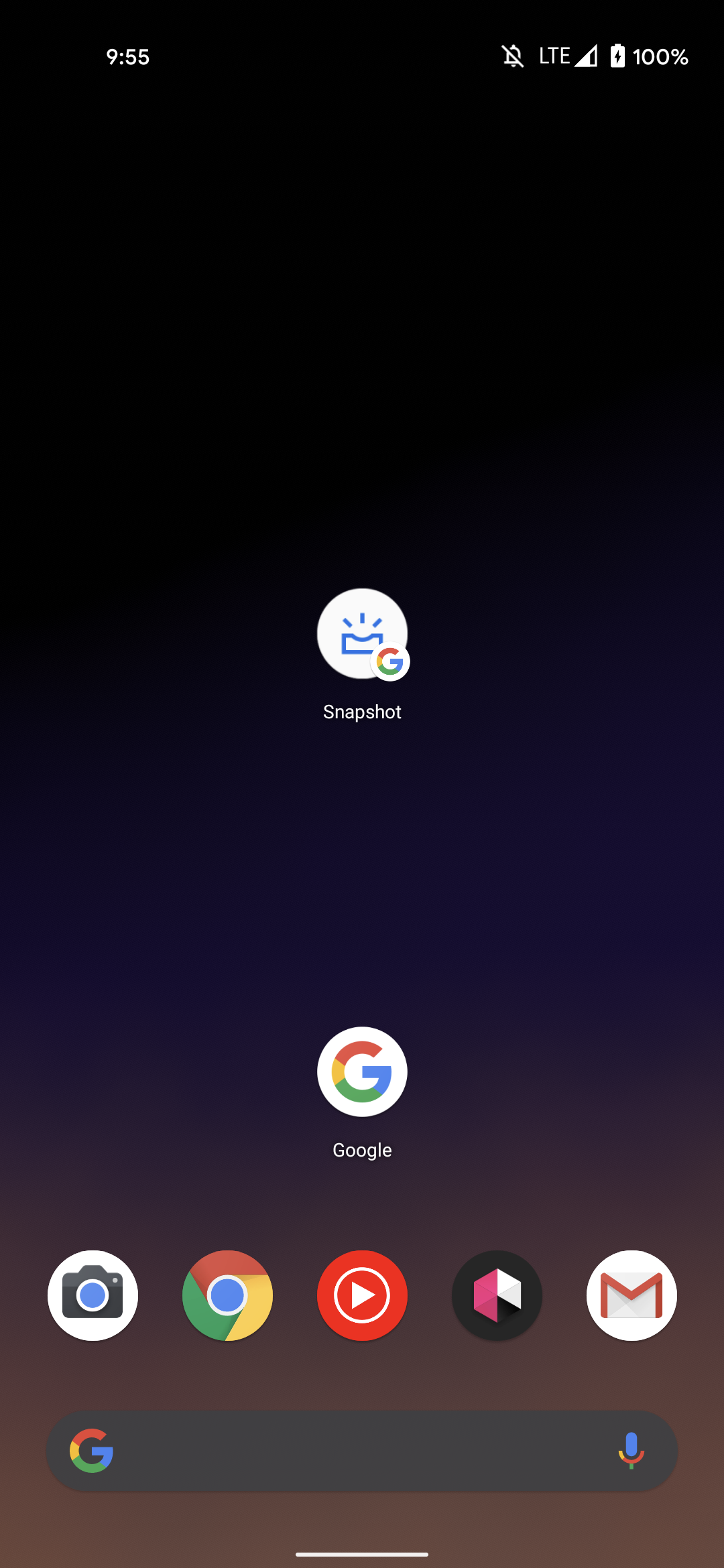This image depicts a phone screenshot with a predominantly black background. In the upper left corner, the time is displayed as 9:55. Moving to the right, there is a crossed-out bell icon indicating that notifications are silenced. Next to it, the LTE icon denotes the network status, followed by a three-quarter full signal strength icon. Further to the right, there is a battery icon showing a full charge at 100%.

Centered prominently is the word "snapshot," accompanied by a circular icon containing a distinct shape. At the bottom of the screen lies the Google logo, situated above a row of five app icons. These icons include a camera, Google Chrome, YouTube, Gmail, and one unrecognized icon.

Below this row, there is a search bar featuring the Google "G" logo with its characteristic red, orange, green, and blue colors. At the end of the search bar, there is a microphone icon for voice input. The entire screen has a black background extending three-quarters of the way down.